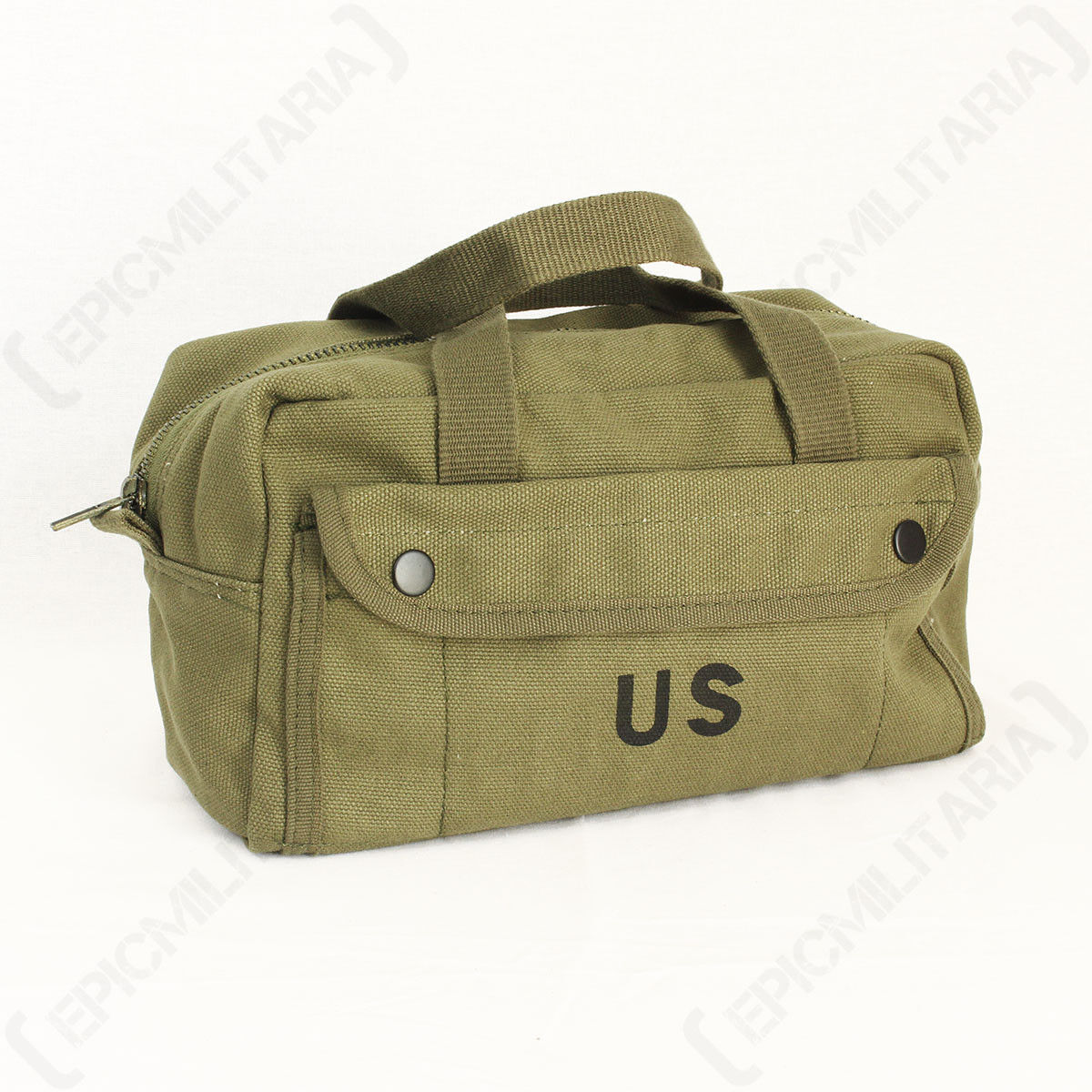This image showcases a green canvas U.S. Army surplus bag on a white background. The central focus of the photograph is the bag, which features the letters "U.S." prominently displayed on the front. The bag includes a main compartment with a green zipper running across the top, complemented by two sturdy handles for easy carrying, similar to a duffel bag. Additionally, there is an exterior pocket on the front, fastened with two black buttons, and a smaller pocket on the far left-hand side for extra storage. The image is overlaid with multiple watermarks that read "Epic Militaria" enclosed in brackets, hinting at the source being a stock image or a promotional photo from the company. The texture of the bag is green canvas, and it could potentially serve various purposes, from carrying toiletries if small, to clothing and gear if larger.